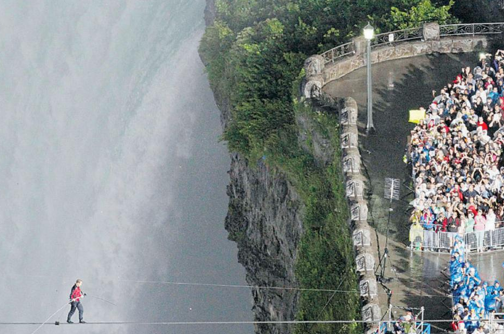This photo captures a high-angle view of renowned tightrope walker Nick Wallenda traversing a tightrope at Niagara Falls. Clad in a red shirt and black pants, Wallenda is positioned in the bottom left of the image, gripping his balancing rod as he focuses on his footing. The tightrope stretches beneath him, while a safety wire runs above. The majestic Niagara Falls serve as a dramatic backdrop, with their green surroundings and white rapids prominently displayed. To the right, a substantial crowd of onlookers stands on a stone platform, separated from the falls by a protective barrier, which is interspersed with a couple of streetlights. The scene is dynamic and enthralling, showcasing a breathtaking blend of natural wonder and human daring.